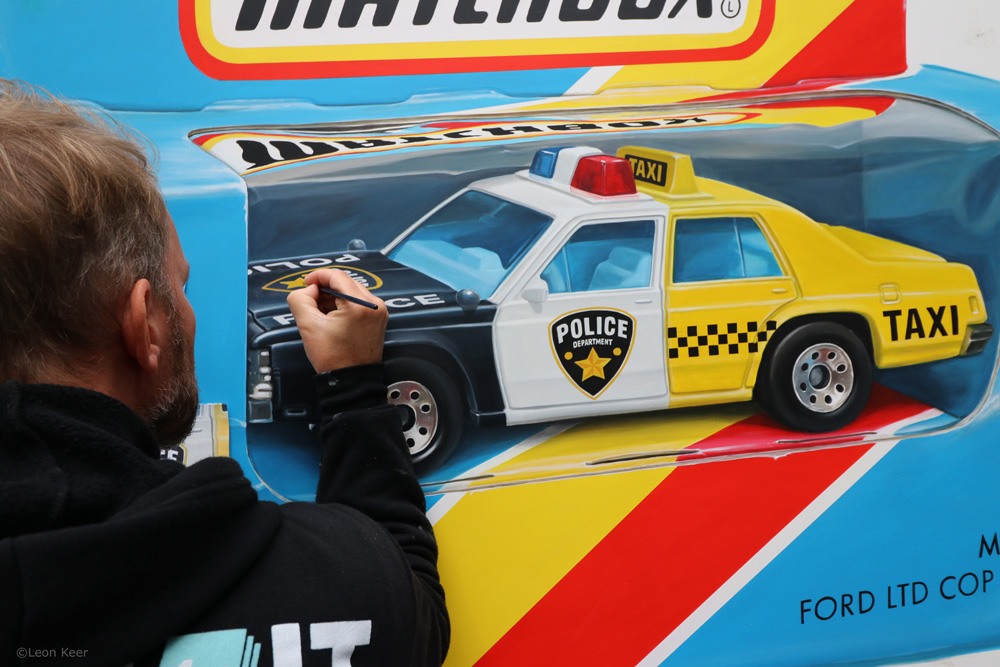In this photograph, a highly detailed and oversized Matchbox car is being autographed. The toy car, encased in a large box with a clear plastic window, features a unique design: the front half is styled as a black and white police car, complete with a badge and labeled "Ford LTD COP," while the back half is a yellow and black taxi cab. The box itself is vibrant with turquoise blue, red, yellow, and white colors, prominently displaying the Matchbox logo in black text. Positioned in the bottom left corner of the image, a person wearing a black hoodie with obscured white text and graphics on the back, can be seen signing the car with a black pen. The photograph's background includes a white wall, and the image is marked with semi-transparent light gray text that reads "copyright Leon Kier" in the bottom left corner.